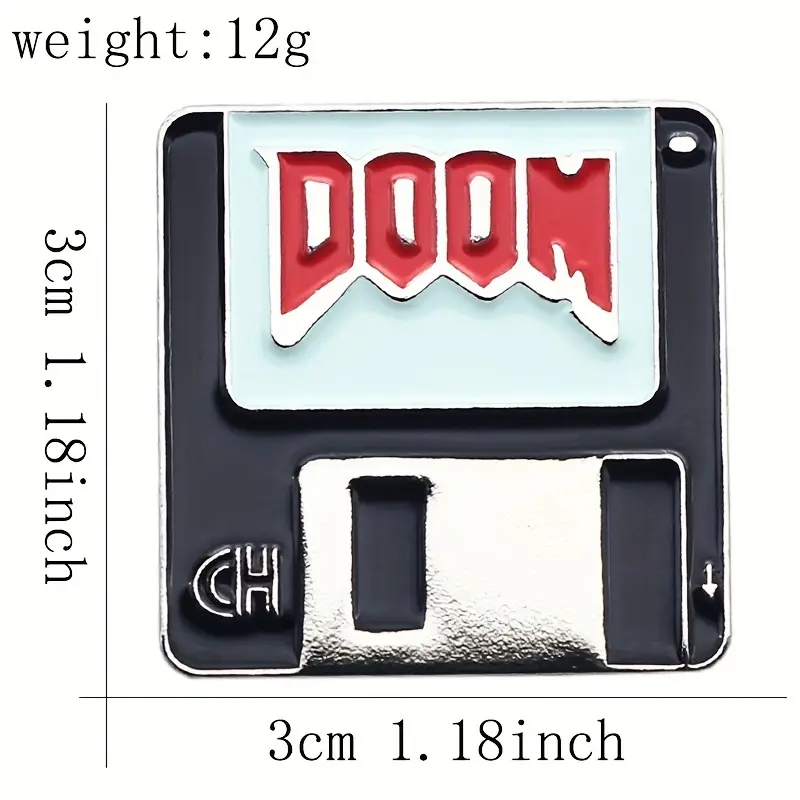This image features a metallic plate intricately designed to resemble a classic floppy disk, set against a pristine, solid white background. The plate itself is predominantly black, emulating the floppy disk's characteristic appearance. At the bottom of the plate, a silver sliding mechanism adds an authentic touch. Positioned near the top, a white label carries bold red text that reads: "Zoom". Additional details printed on the plate in red text include its weight, labeled as "12g", and its dimensions: "3 centimeters (1.18 inches) by 3 centimeters (1.18 inches)". These precise measurements and the clear, high-contrast color scheme make this object both visually striking and reminiscent of the iconic floppy disk.